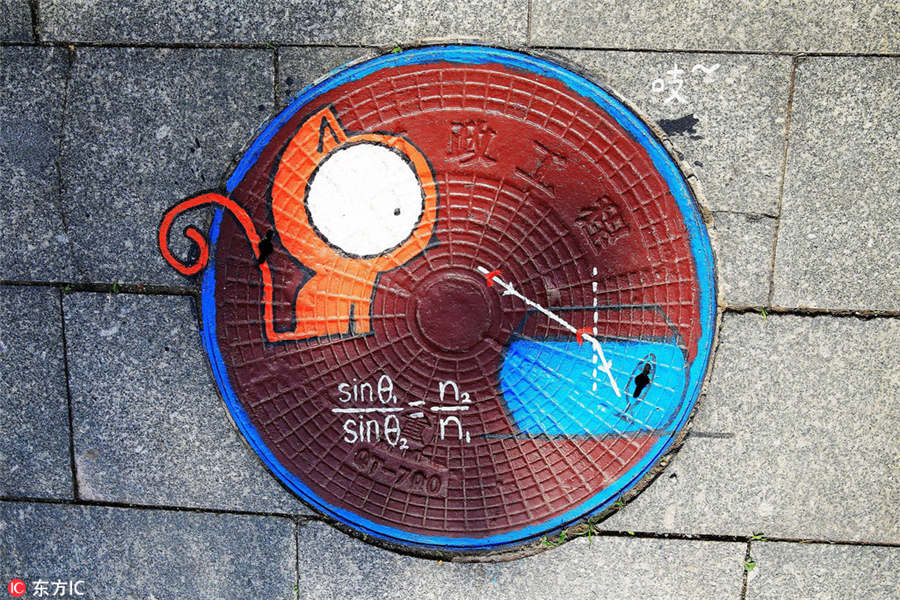This image is a detailed, painted manhole cover situated on a brick or cobblestone sidewalk. The manhole cover is predominantly a dark, almost blood-red color with a light blue border. On the cover, an orange cat with an exaggerated, large white eye is depicted in a distinctive cartoon style. The cat appears to be interacting with or looking at a small, unclear blue figure beneath it. Additionally, there is a mathematical equation inscribed at the bottom of the cover, reading "sin θ1 over sin θ2 equals n2 over n1." There's a light blue rectangle nearby this equation. Along the bottom left edge of the circle, there's some writing, including a red circle with what appear to be Asian characters followed by "IC." The image captures the intricate design set against the textured gray of the sidewalk, which may be either cement or brick.